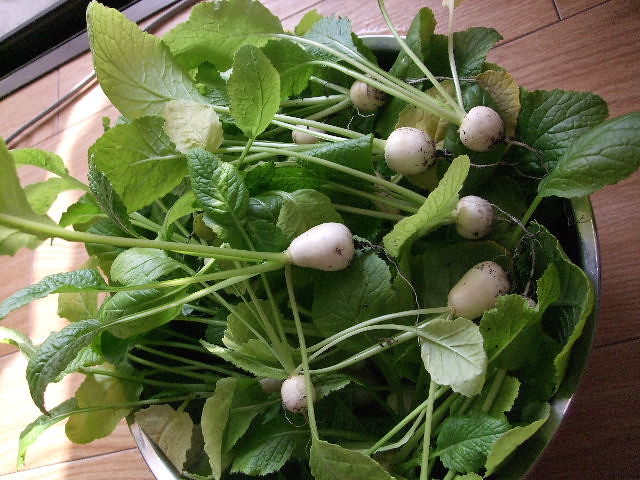This image captures a bird's-eye view of a round, silver metal bowl overflowing with freshly harvested white radishes, complete with their green stalks and leaves still attached. The radishes, covered with a bit of dirt, suggest they were recently pulled from the ground. This abundance of radishes is placed on a brown surface, likely a wooden floor, given the visibility of what appears to be the base of a door in the top left corner of the photograph, adding a hint of domesticity to the scene. The photo's backdrop is consistently brown, echoing the earthy and rustic theme of the freshly picked vegetables.